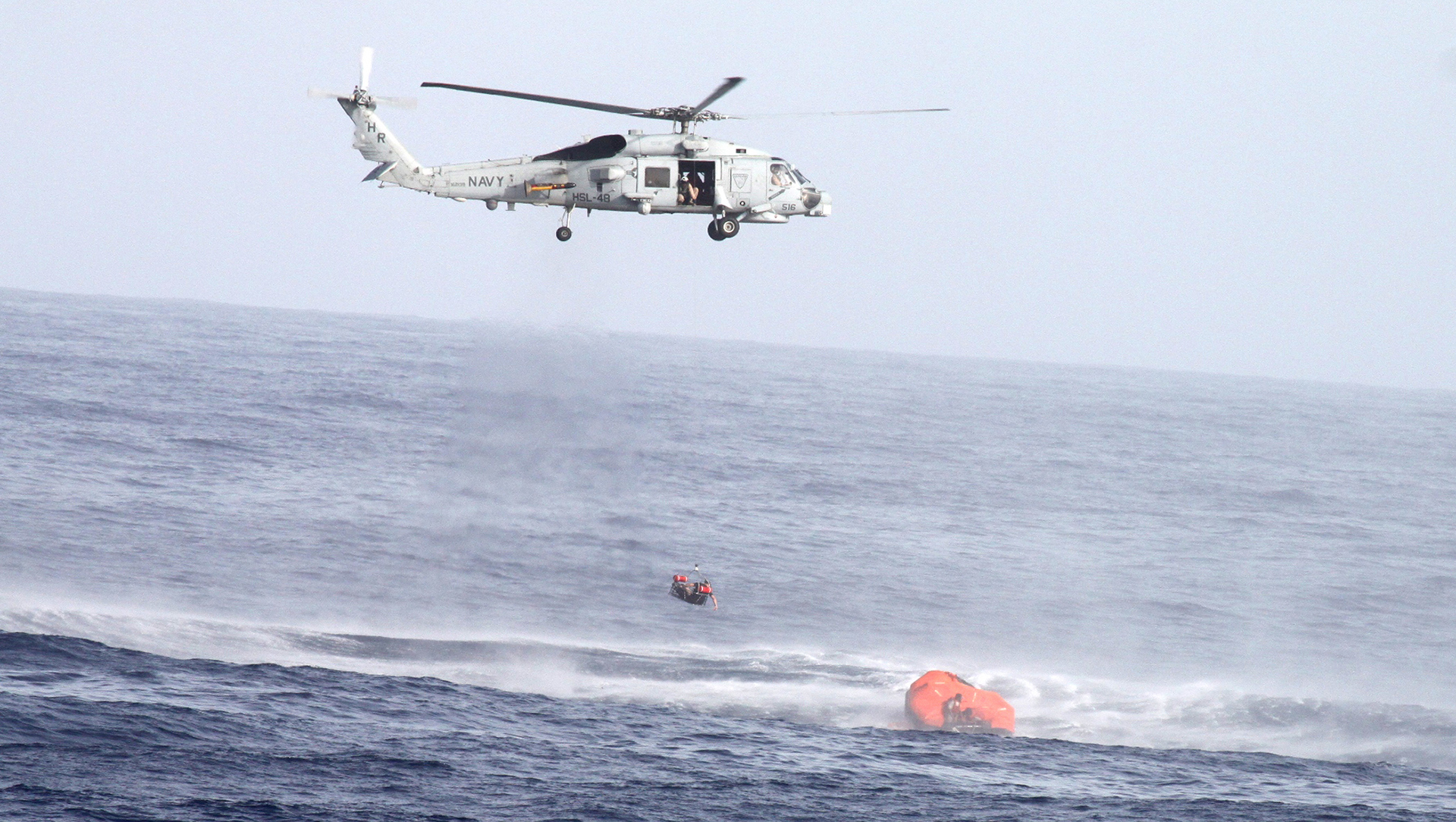This detailed photograph captures an intense naval search and rescue operation over a tumultuous ocean. In the foreground, dark bluish-gray waves with frothy white tips crash violently, indicating rough seas. The water's hue transitions to a misty light gray as the view recedes into the horizon, which is tilted slightly higher on the left.

Dominating the top portion of the image is a white Navy helicopter, flying towards the right under a hazy sky that blends shades of blue and light gray. The helicopter, captured with its three black blades seemingly frozen by a high shutter speed, hovers with its landing gear extended. The open side door reveals personnel inside, and ropes dangle down towards the ocean below.

Beneath the chopper, situated in the more agitated waters, an orange rescue raft can be seen with tiny silhouettes of people aboard, suggesting they are awaiting rescue. There also appears to be another section farther away, showing hints of black and red amidst the waves, possibly related to the rescue effort. This photograph vividly conveys the urgency and peril of the rescue mission in such harsh marine conditions.